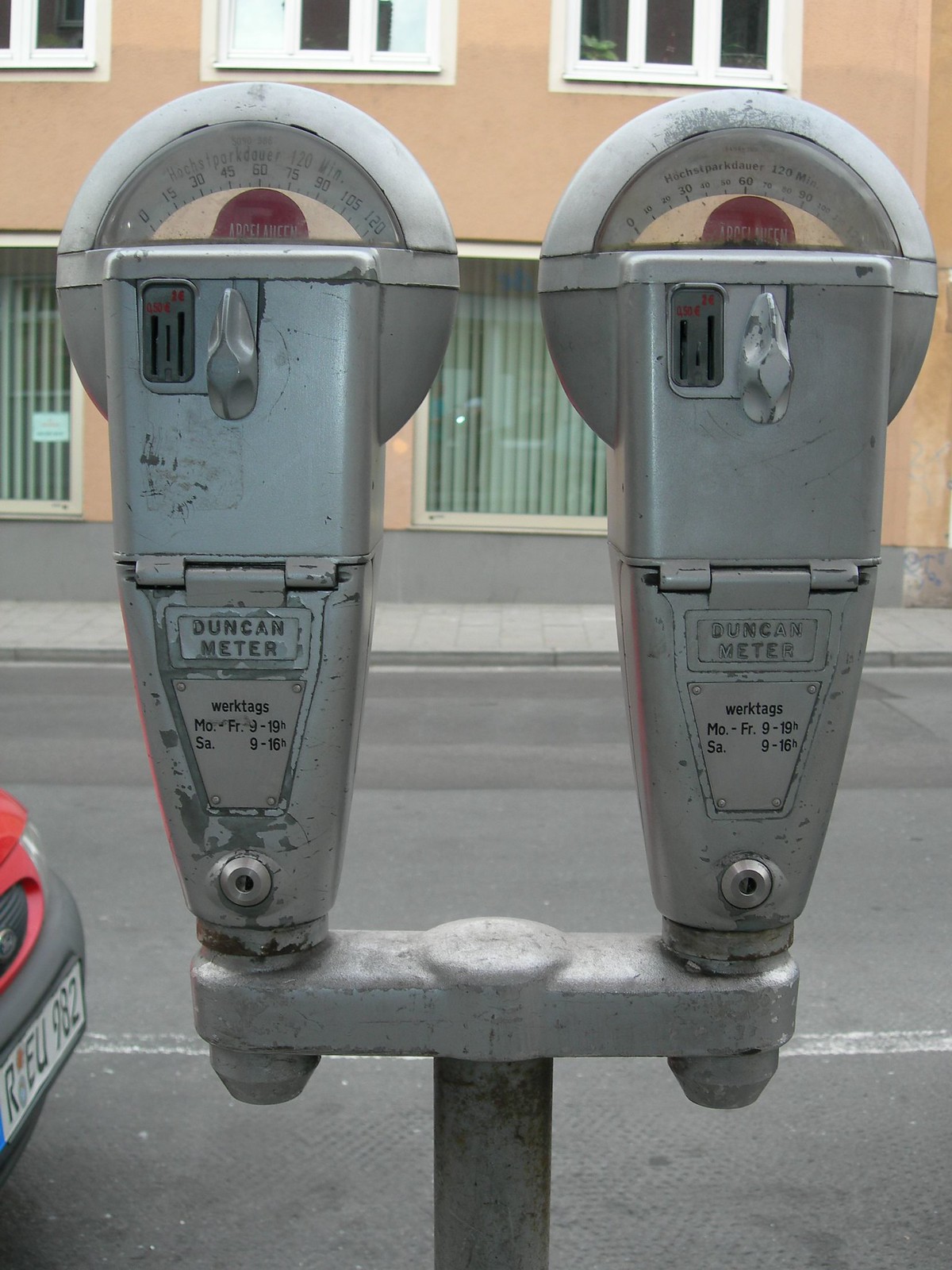The image captures two old, silver-colored parking meters mounted on a heavy-duty metal pole with a T-bracket at the top. Each meter, branded "Duncan Meter" in raised lettering, features coin slots for different-sized coins and dials marked from 0 to 120 minutes. Red flags indicating expired time are visible through the glass domes. Below the brand name, the operational hours are specified in German: Monday to Friday from 9 to 19H and Saturday from 9 to 16H. In the background, a peachy beige or tan-colored building with brownish-yellow hues stands, adorned with large windows framed in white and equipped with vertical blinds, with at least one showing a green plant. Below the building’s windows, a gray sidewalk leads to the black-topped street, which sports a faded white line. On the left side of the image, partly visible, is a red car with a black bumper and a German license plate reading REU 982. The scene suggests a typical European city street. Subtle details include the light gray of the concrete, minor scratches on the meters, and the tactile texture transitions between the sidewalk and the road.